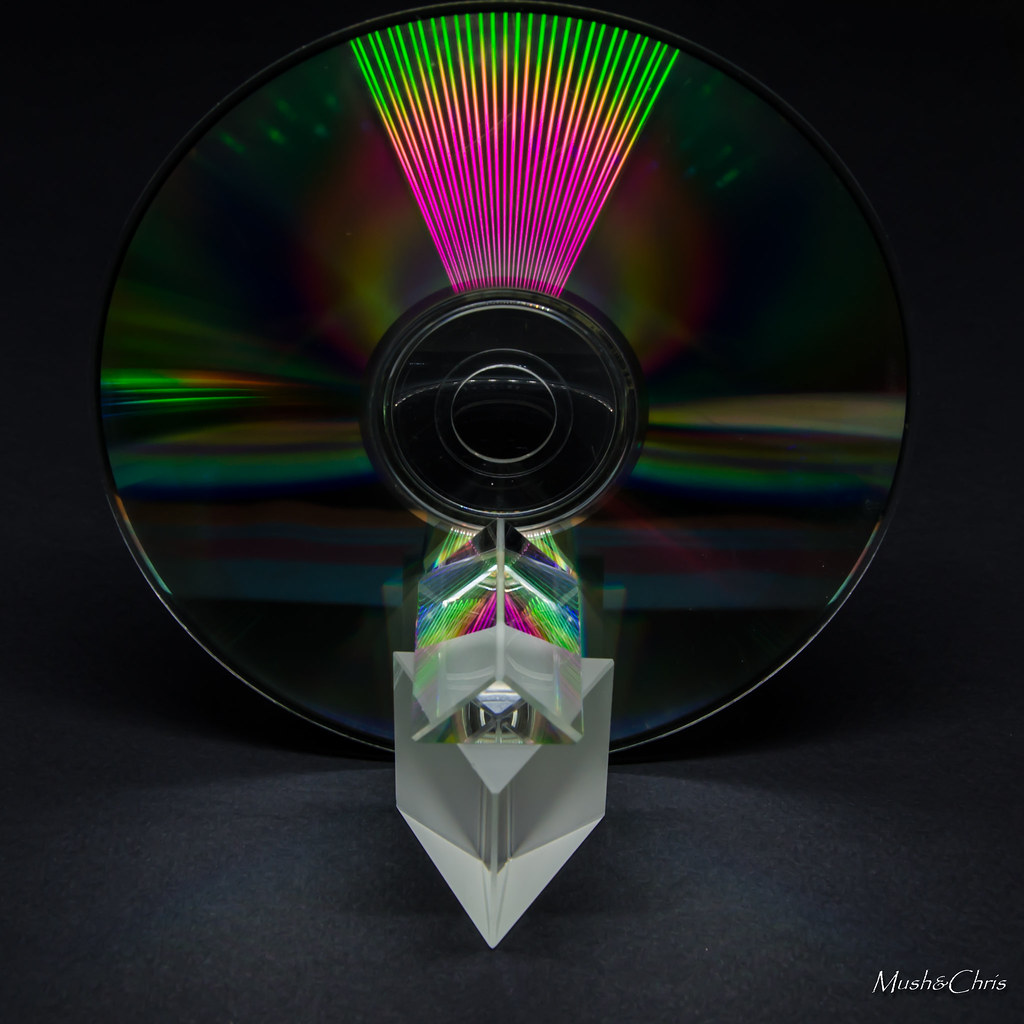The image is a photograph featuring a compact disc held vertically on a dark background, with the names "Mush and Chris" signed in white lettering in the bottom right corner. The disc is elevated by two prisms: one is a half-rectangular prism and the other a triangular prism. Neon-colored rays radiate from the top of the disc, transitioning from neon pink to neon orange, and finally to neon green. The center of the disc is clear, amplifying the diffraction effect that spreads out the light into various neon colors. Below the center and the radiant rays are additional vibrant neon rays in blue, green, and pink along with a white plastic object accented with chrome, near the disc. The reflective surface of the disc and the prisms create a spectral display of colors, artfully enhanced by a digital or artistic overlay, making the entire light spectrum visible against the dark backdrop.